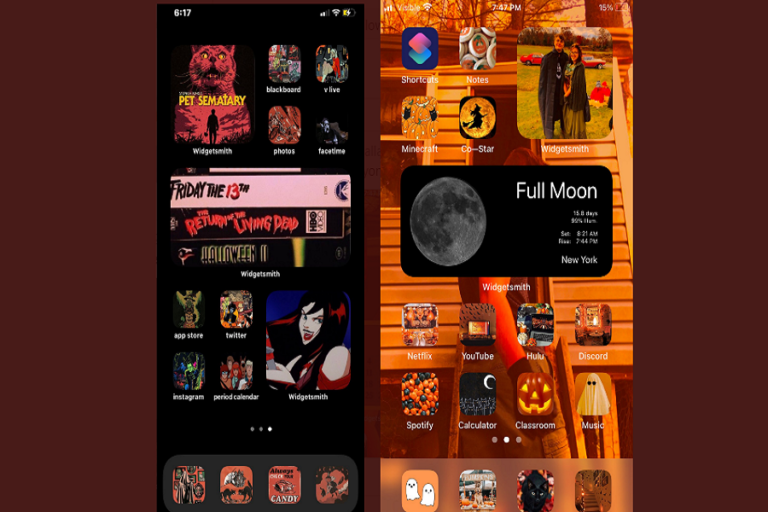This image consists of two smartphone screenshots placed side by side, showcasing different thematic content. 

The left screenshot features a predominantly black background filled with several small square images depicting scenes from various horror movies. Among these movie stills, notable titles include "Pet Sematary." Below this, there is a prominent pink rectangle with the title "Friday the 13th" displayed. Further down, another black rectangle with red text reads "Return of the Living Dead." Additional horror movie scenes and titles populate the remainder of this screen, creating an engaging collage of classic horror references.

The right screenshot showcases a more festive, Halloween-themed aesthetic with shades of orange permeating the background, which appears to be an altered photograph of a house. In the center of this screenshot, a black rectangle with rounded corners prominently displays the text "Full Moon" in white font. To the left of this text, there is an image of the moon. Below this central section, there are various thumbnail images indicative of Halloween traditions, including a jack-o'-lantern, assorted Halloween candy, and a ghost costume with two black eyes.

Together, these screenshots provide a vivid juxtaposition of horror movie motifs and Halloween celebration imagery.